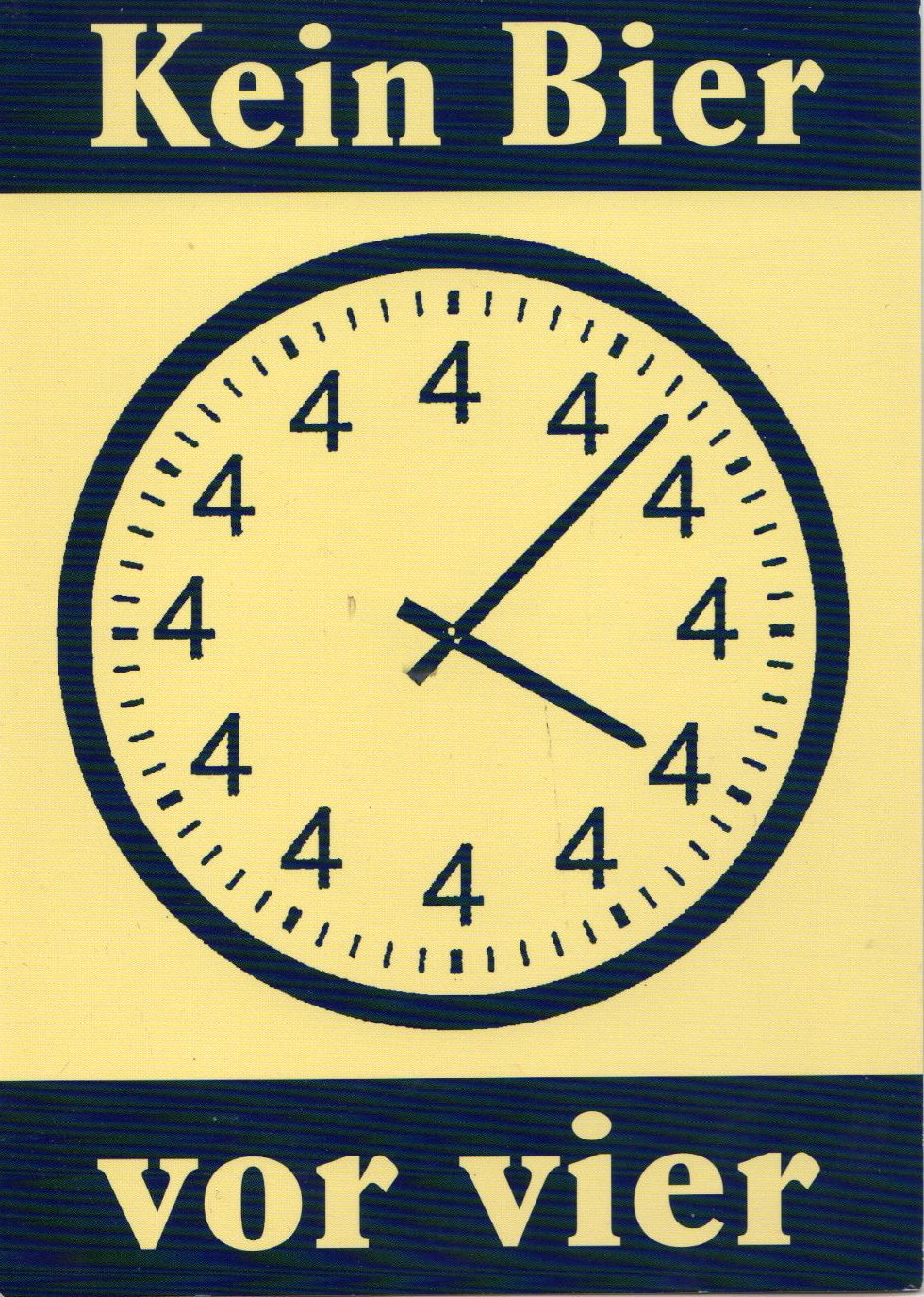The advertisement image has a striking design dominated by a central clock where all the usual numbers (1 through 12) are replaced by the number 4. The clock, featuring black hands and markings, is set against a vivid yellow background. A black border frames the top and bottom of the image. The top black banner contains the text "Kein Bier" in yellow, and the bottom black banner reads "VOR VIER," also in yellow. The small hand of the clock points to one of the number fours on the right side, while the large hand sits between two of the fours. This clock, with its repetitive numeric design and bold color contrast, serves as the focal point of the advertisement.